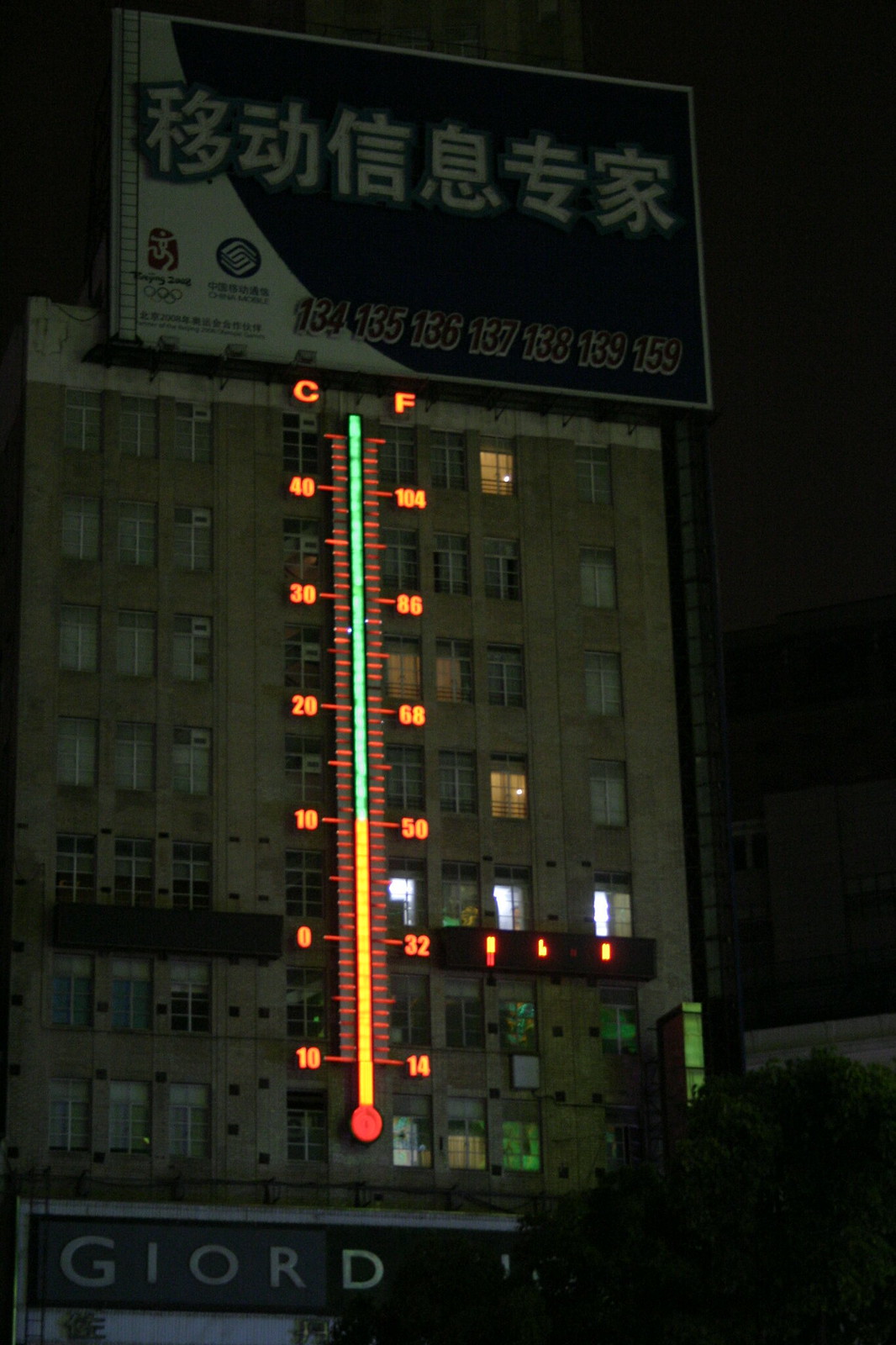This nighttime photograph captures the side of an aged, New York City-style brick building, located in China. Dominating the scene is a large, illuminated billboard featuring Chinese characters, the colors of which are somewhat obscured in the dim light, possibly being either black and white or blue and white. Beneath the characters, a series of numbers ranging from 134 to 159 are prominently displayed.

The building itself stands at nine stories tall, and a striking feature is the digital thermometer that extends vertically across its facade. The thermometer displays the temperature in both Celsius and Fahrenheit, currently showing 50 degrees Fahrenheit (10 degrees Celsius). The scale on the thermometer ranges from 10 degrees Celsius to 50 degrees Celsius.

At street level, there's a storefront with a partial sign visible due to a tree obstructing the view. The visible letters spell out "G-I-O-R-D," suggesting the name of the business. The building shows signs of life, with a few windows illuminated by green and regular fluorescent lights. The overall composition highlights the contrast between the traditional structure and the modern digital elements, set against the quiet backdrop of a Chinese city at night.